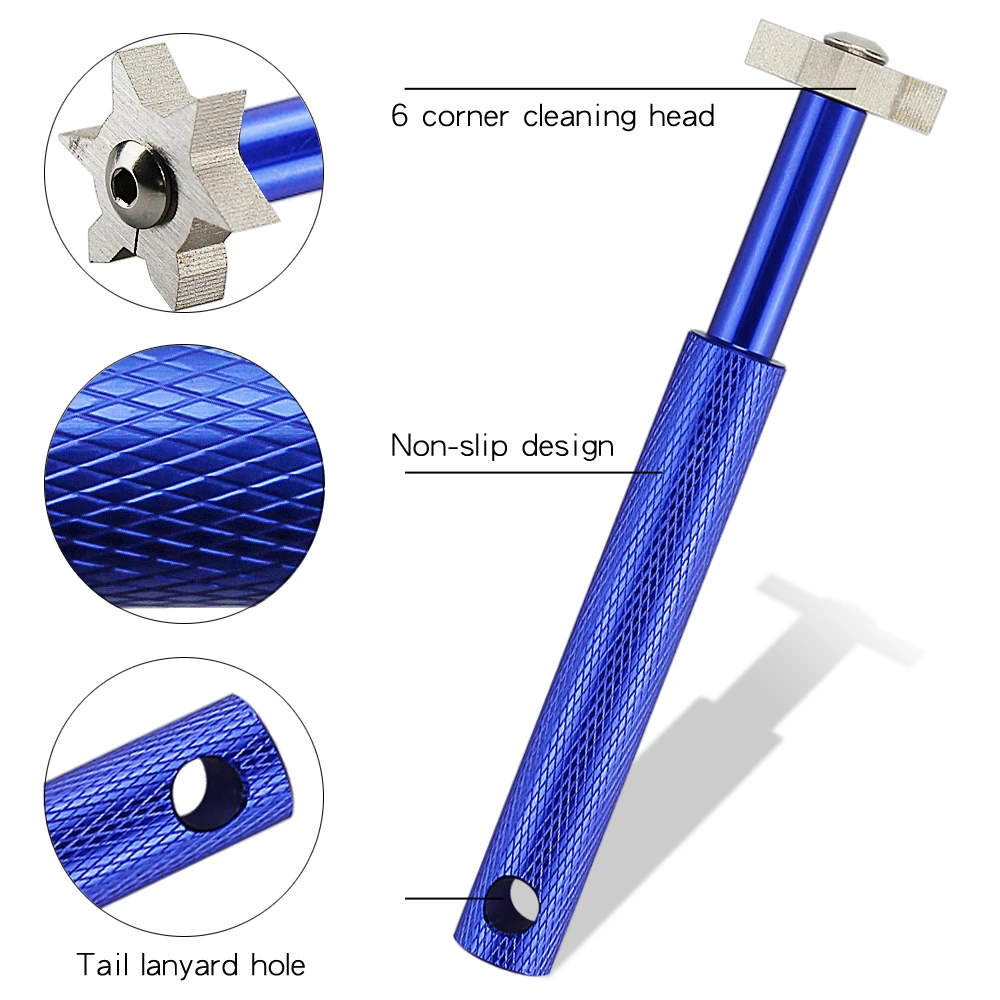This image features a detailed computer-generated representation of a cleaning tool set against a white background. The tool, prominently positioned from the center bottom to the upper right corner, is comprised of a handle and a cleaning head. The handle is a smooth blue metal rod with a distinct non-slip design created by diagonal ridges for better grip. At the bottom of the handle, there is a tail lanyard hole intended for attaching a lanyard. The cleaning head, which is silver and star-shaped with six sharp corners, is fixed to the handle with a bolt. The image includes three inset circles showcasing close-ups of notable features: the six-corner cleaning head, the non-slip handle design, and the tail lanyard hole. The tool casts a shadow to the left, indicating the light source's direction. Text at the top of the image highlights the product features, such as the "Corner Cleaning Head Non-Slip Design." This tool appears to be used for tasks like grout removal or similar cleaning activities.